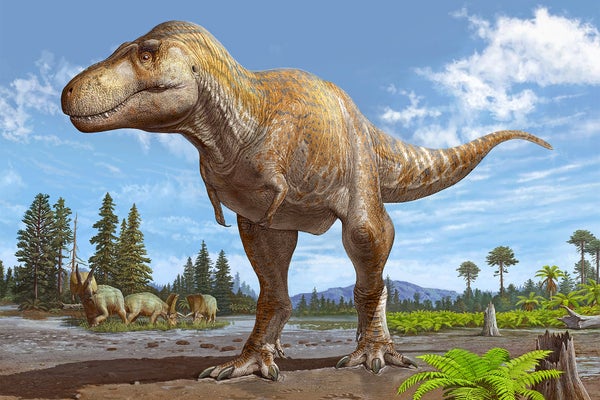This highly detailed, digitally-rendered image appears to originate from a video game, movie, or computer program, evoking a prehistorical setting. The scene is set outdoors and transports viewers to an ancient time. The ground is primarily composed of mud interspersed with rocks, creating a rugged terrain. To the right side of the foreground, several small fern plants are visible, with a prominent one situated in the middle. A sturdy tree trunk stands adjacent to this central fern. In the background, a majestic range of mountains looms, providing a dramatic backdrop to a dense expanse of tall trees. The forest comprises a mix of pine trees and other varieties characterized by tall trunks with foliage concentrated at the top.

Dominating the left side of the scene, three dinosaurs graze near the tree line. They are herbivorous creatures with elongated heads, adorned with two prominent horns at the front, and supported by four sturdy legs. The image's central and most striking subject is a towering Tyrannosaurus rex positioned at the forefront. This T. rex is depicted with a massive head, its closed mouth partially exposing fearsome teeth. It has notably short, stubby arms contrasting with its long, powerful legs and a substantial, robust tail, emphasizing its formidable presence in this prehistoric landscape.